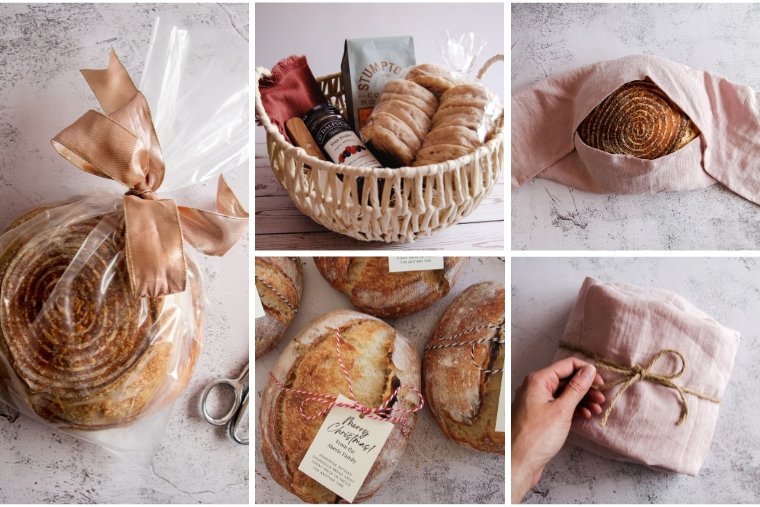The image is a detailed collage of five photos showcasing various gourmet breads, neatly wrapped and presented, ideal for gifting. On the left-most side, there is a clear cellophane package containing a round loaf of sourdough bread decorated with concentric circles, sealed with a gold bow and paired with a set of metal scissors on a white and gray marble countertop. Above, a tan woven gift basket sits on a wooden surface, filled with an assortment of sweetbreads, a gray coffee bag, some cookies, and a knife with a wooden handle. Below this, three round loaves of bread are individually wrapped in clear cellophane and tied with a red and white string, each adorned with a "Merry Christmas" tag. In the upper-right corner, another loaf similar to the sourdough is wrapped in a white linen cloth, resting on a gray and white marble background. Lastly, in the lower right, a person's hand is seen either tying or untying a package wrapped in white linen and twine, also set against the same marble backdrop. The collage beautifully captures the artisan nature of the breads, with each element meticulously detailed and thoughtfully arranged.